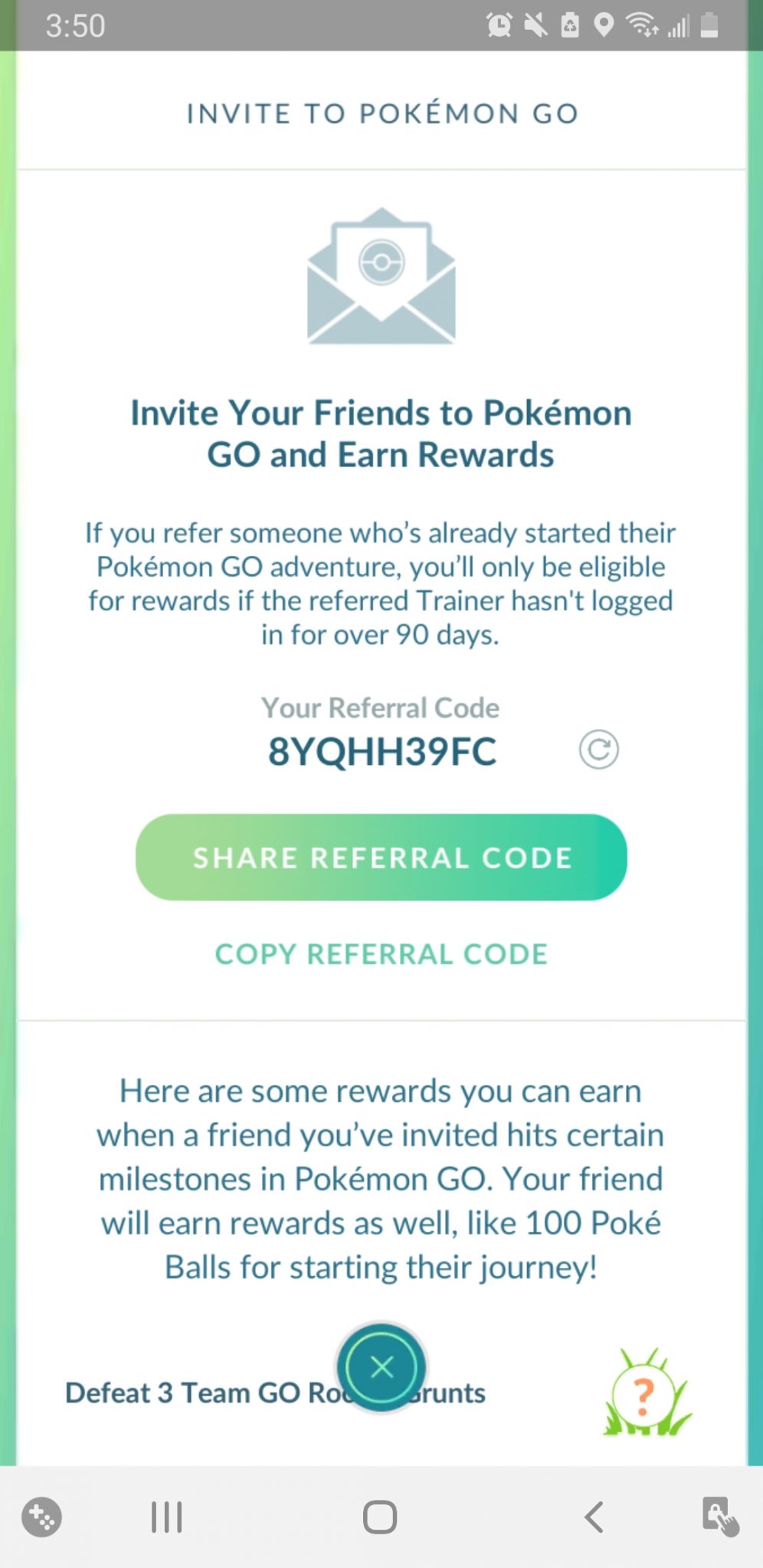This screenshot showcases a mobile application interface for inviting friends to join Pokémon GO. At the top part of the screen, a translucent black bar displays white icons on the top right. Below the bar, the main body of the page is predominantly white with two thin gradient columns on either side. The left column transitions from lime green at the top to bluish green at the bottom, while the right column features a gradient from greenish blue at the top to teal at the bottom.

Centrally placed at the top of the page, blue text in all caps reads "INVITE TO POKÉMON GO." Directly beneath this heading is a thin green line. Below the line, an icon of a blue envelope with a white stylized Pokémon card emerging from it is centered. Under this icon, two lines of blue text state, "INVITE YOUR FRIENDS TO POKÉMON GO AND EARN REWARDS."

Following this, a paragraph of smaller blue text elaborates, "IF YOU REFER SOMEONE WHO'S ALREADY STARTED THEIR POKÉMON GO ADVENTURE, YOU'LL ONLY BE ELIGIBLE FOR REWARDS IF THE REFERRED TRAINER HASN'T LOGGED IN FOR OVER 90 DAYS."

Beneath the paragraph, light gray text indicates, "YOUR REFERRAL CODE," followed by the referral code itself in all caps blue text, "8YQHH39FC." To the right of the code, there's a light gray refresh icon encircled by a light gray border.

Lower down on the page, a button with a gradient transitioning from lighter green on the left to bluish green on the right reads "SHARE REFERRAL CODE" in all caps white text. Finally, at the bottom of the interface against the white background, blue text in all caps reads "COPY REFERRAL CODE."